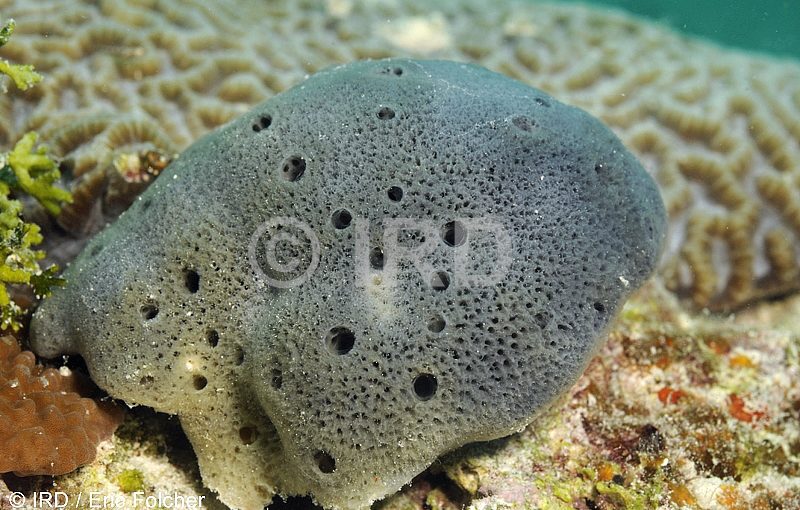This underwater photograph, taken by IRD (copyright IRD / Eno Fulcher), showcases a detailed and textured scene of marine life. The main subject is a gray piece of coral in the foreground, characterized by numerous holes and a highly textured surface. Behind it, there is a substantial piece of brain coral, resembling a thick pancake with a worm-like tan surface. To the left, tree-style green coral and a burnt orange anemone add vibrant touches to the scene. The ocean floor is a colorful mosaic of browns, greens, yellows, and oranges. The water appears blue, framing the intricate details of the marine organisms. A ghosted white watermark reading "IRD" is visible in the photograph.